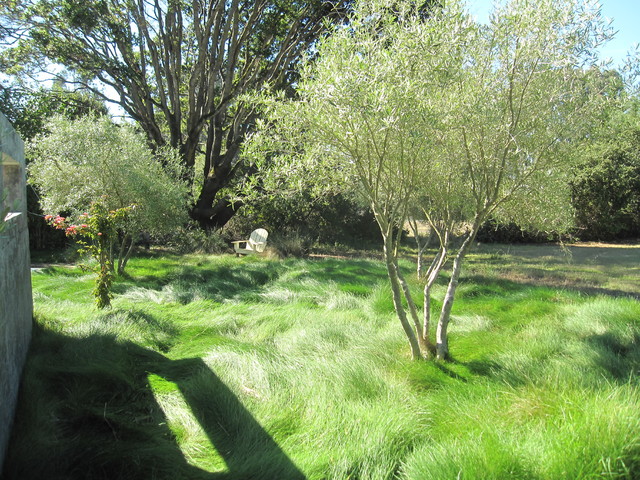An intricate backyard scene is captured in this photo featuring an expanse of tall, verdant grass that appears untrimmed for several months, lending a wild, natural appearance. Nestled in this lush greenery are various trees, including a few short ones with white limbs and faded green canopies, and a towering tree with multiple trunks located towards the left background. Amidst the tall, flowing grass stands a white Adirondack chair with wide wooden armrests, subtly weathered and positioned under the shade of the largest tree. On the far left edge, a concrete structure with an open, glassless window casts a shadow over part of the lawn, adding a rustic touch to the scene. The grass, though slightly dry in areas, maintains a vibrant green hue, indicative of its overall health.